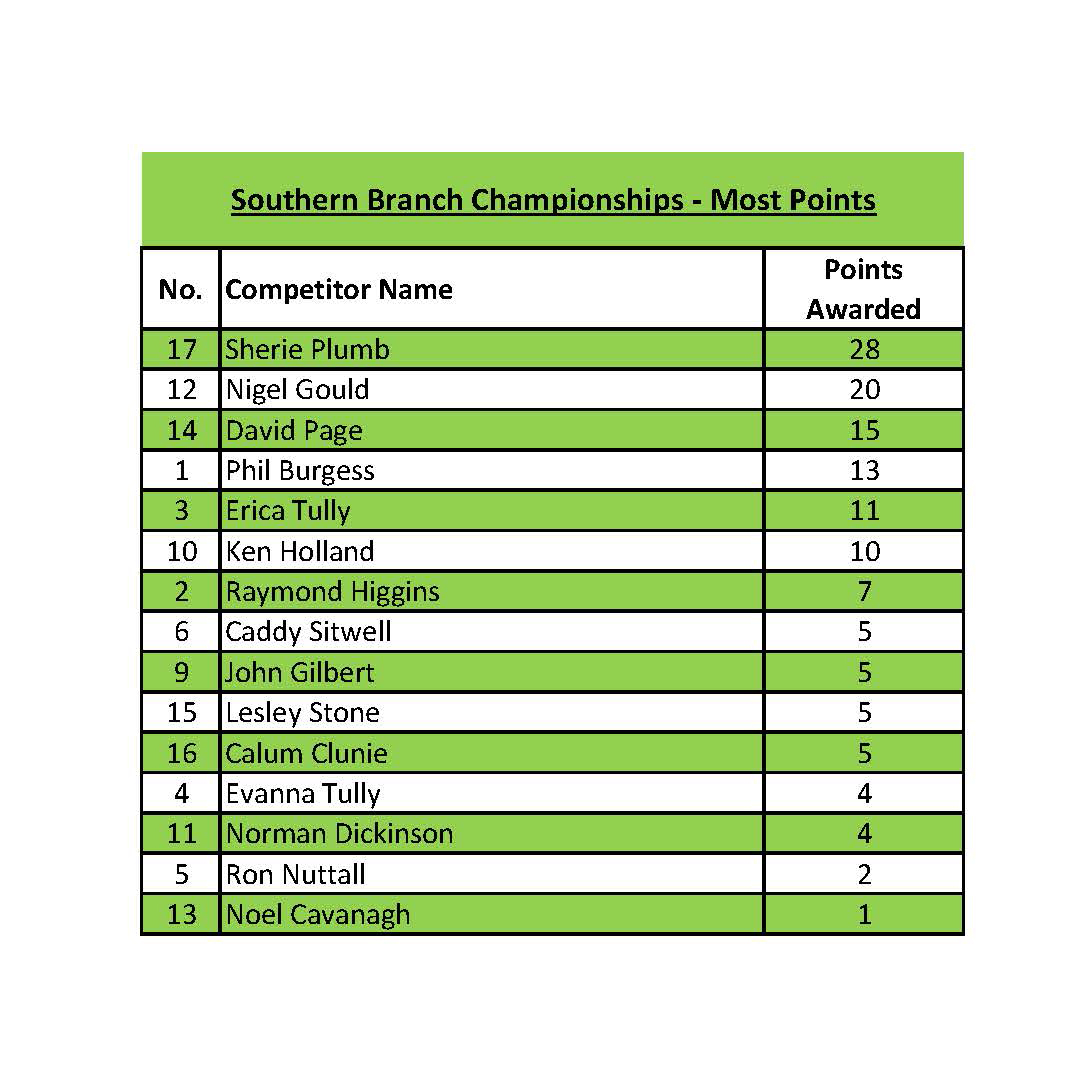This image is a detailed chart depicting the Southern Branch Championship rankings based on points awarded. At the top of the chart, a green header prominently features the title, "Southern Branch Championship – Most Points," in black letters with a black line underneath. The chart is organized into three columns labeled “NO.,” “Competitor Name,” and “Points Awarded.” Each row alternates between white and blue rectangular bars for contrast. The competitors are ordered by their points, from the highest to the lowest.

In ascending numerical order, the competitors and their points are as follows: 
- No. 17 Sherry Plum with 28 points
- No. 12 Nigel Gould with 20 points
- No. 14 David Page with 15 points
- No. 1 Philip Burgess with 13 points
- No. 3 Erica Tully with 11 points
- No. 10 Ken Holland with 10 points
- No. 2 Raymond Higgins with 7 points
- No. 6 Caddy Stillwell with 5 points
- No. 9 John Gilbert with 5 points
- No. 15 Leslie Stone with 5 points
- No. 16 Callum Conley with 5 points
- No. 4 Evan Antolley with 4 points
- No. 11 Norman Dickinson with 4 points
- No. 5 Ron Nuttall with 2 points
- No. 13 Noel Kavanne with 1 point

The design efficiently compares competitors based on their point totals, providing a clear visual representation of their rankings.